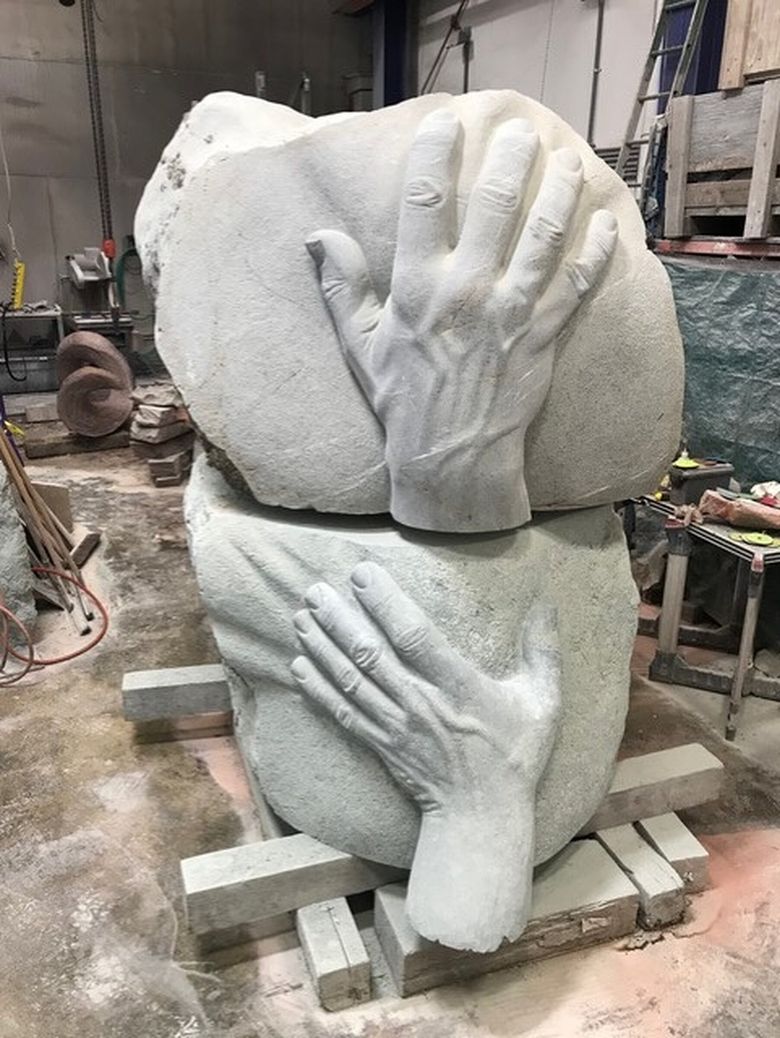The image depicts a detailed and visually impactful stone sculpture within a workshop setting. The scene is set inside a shop characterized by dark gray metal walls and scattered equipment on numerous small tables in the background. On the right side, a large white bay door and a long silver ladder are prominent. In the foreground, two substantial pieces of white rock catch the eye, intricately carved with large, lifelike hands that appear to grasp the rocks from top to bottom. These hands are remarkably detailed, showcasing knuckles, veins, and fingernails, expertly rendered to enhance their realism. The rocks rest on a platform composed of cement blocks and wooden posts, all situated on a concrete floor dusted with light pink and white powder, likely residue from the sculpting process. The foreground platform, made of what seems to be marble or stone, underscores the weight and solidity of the sculpture, emphasizing its impressive craftsmanship and scale.